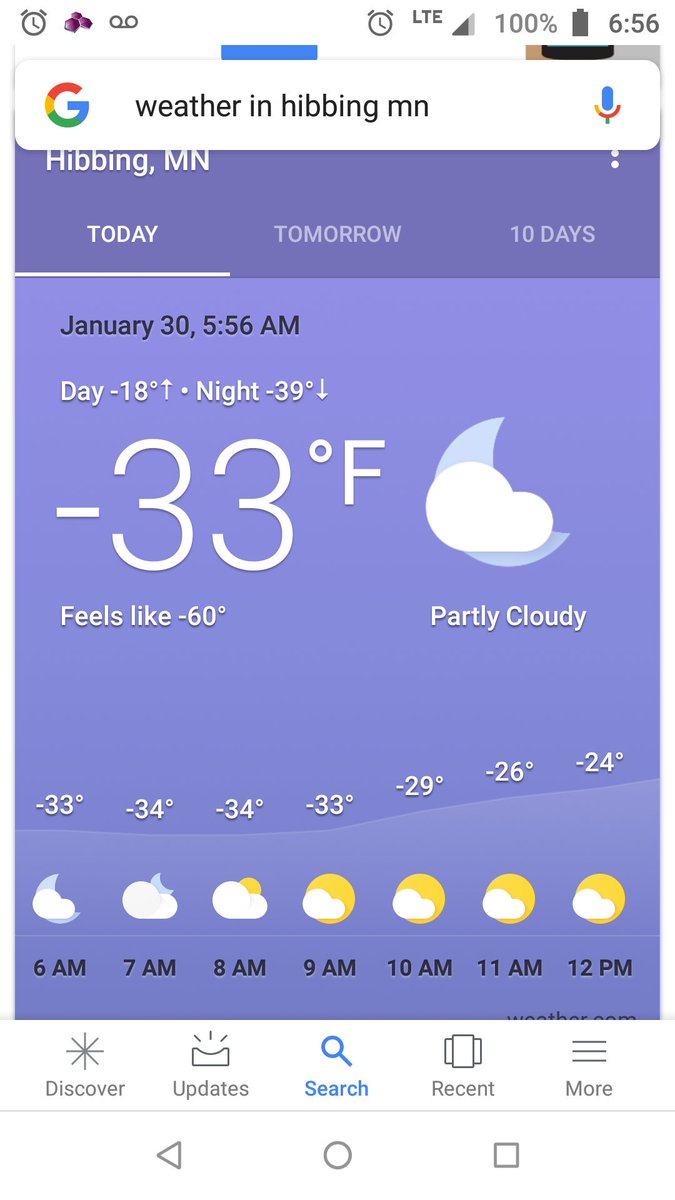A detailed screenshot of a cell phone display shows several distinct elements. At the very top, the status bar displays various icons: an alarm clock, a purple icon resembling grapes, a message indicator, another alarm clock icon, an LTE signal indicator with four out of five bars, a battery icon at 100% charge, and the time displayed as 6:56 AM. 

Below the status bar is a Google search bar with the query "weather in Hibbing, MN," accompanied by a microphone icon on the right. Following this is a header with a purple background indicating the location "Hibbing, MN." Below the header are three tabs: "Today" (selected in white), "Tomorrow," and "10 days."

The weather details for January 30th at 5:56 AM are listed under the "Today" tab. The day's temperatures are highlighted with the daytime high anticipated to be -18°F and the nighttime low plummeting to -39°F. The current temperature is -33°F, with a wind chill making it feel like -60°F. The partly cloudy condition is represented by an icon featuring a cloud and a partial moon.

Further down, there is an hourly forecast section listing times and corresponding temperatures: 6 AM (-33°F), 7 AM (-34°F), 8 AM (-34°F), 9 AM (-33°F), 10 AM (-29°F), 11 AM (-26°F), and 12 PM (-24°F).